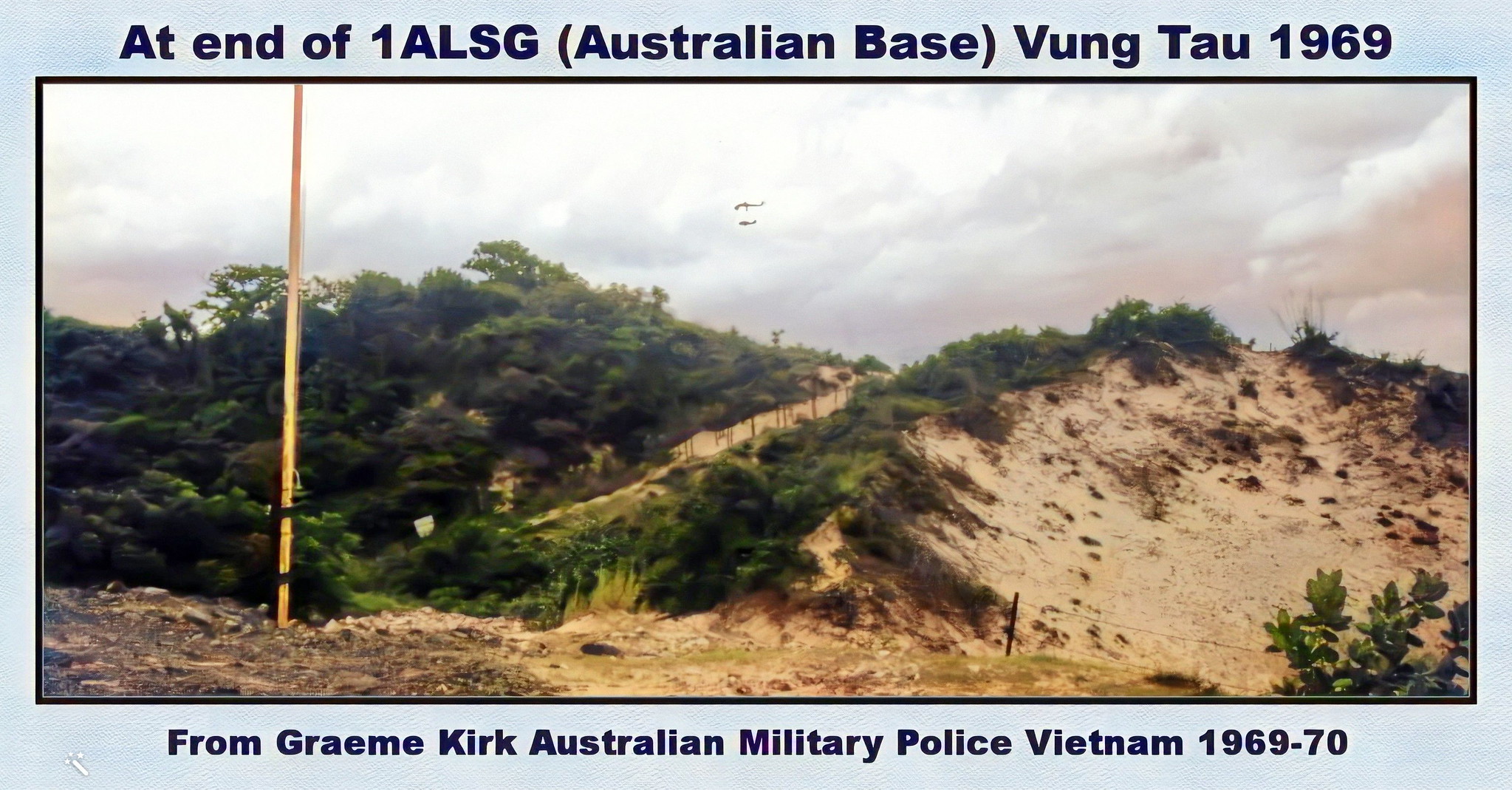This vintage photograph, taken in 1969 at the Australian base 1ALSG in Vung Tau, Vietnam, captures a sandy, hilly terrain characterized by high sand dunes and an abundance of green bushes, brush, and trees. A prominent yellow pole stands on the left side, reaching up to the top of the image. The sky above is clouded, and a helicopter can be seen flying overhead, potentially carrying supplies. The image has an old-looking quality, framed by a dark border with a light blue outer border. The top of the image is annotated in dark blue text with "At end of 1ALSG (Australian Base), Vung Tau, 1969," and the bottom reads "From Graham Kirk, Australian Military Police, Vietnam, 1969-70."